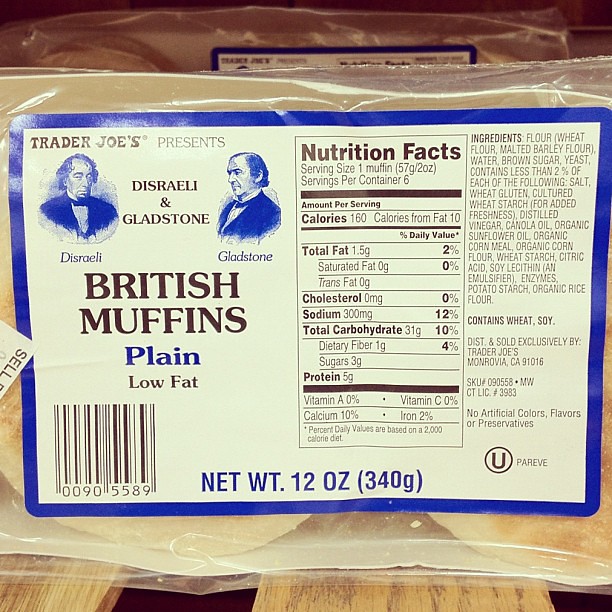The image features a clear plastic package of British muffins from Trader Joe's, sitting upright on a wooden pallet. The package showcases a large, beige rectangular label bordered in navy blue on its front side. Prominently displayed at the top left is the Trader Joe's logo. Below it, two vintage-style portraits of two Caucasian men in suits and bowties—identified as "Disraeli" and "Gladstone"—are visible. In the center, the label reads "Trader Joe's presents Disraeli & Gladstone British Muffins, plain, low-fat." Beneath this, a UPC barcode is located, accompanied by the net weight information: "12 ounces (340 grams)." 

The bottom section of the label includes detailed nutrition facts, indicating that each muffin contains 160 calories and has 10 calories from fat. The nutritional breakdown includes total fat, cholesterol, sodium, total carbohydrates, and protein, along with vitamin A, vitamin C, calcium, and iron content. Additionally, there's a comprehensive list of ingredients such as flour, distilled vinegar, and canola oil, noting that the product contains wheat and soy. The label also features a kosher certification symbol (a "U" inside a circle) and mentions that the product has no artificial colors, flavors, or preservatives.